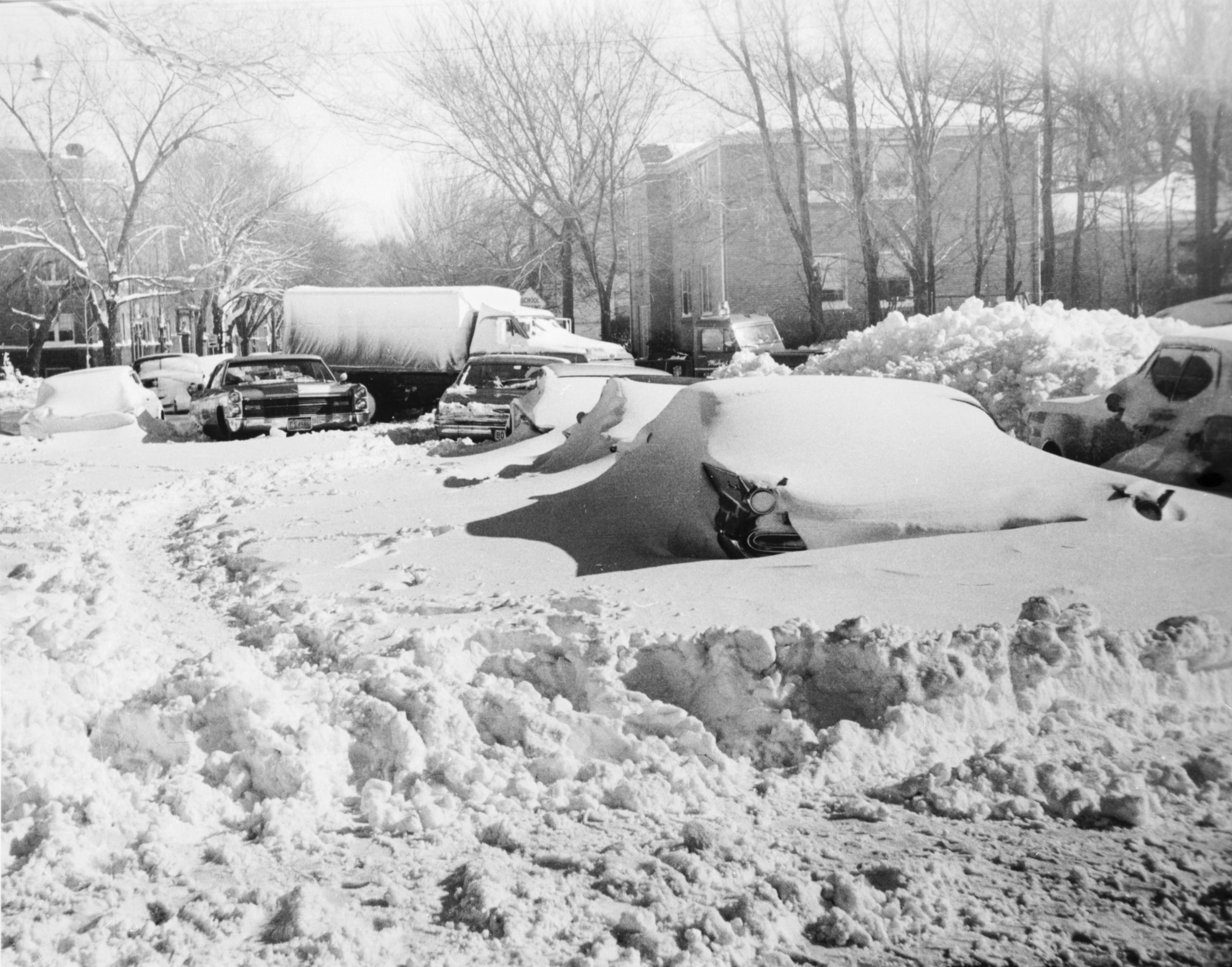The black and white photograph captures the aftermath of a substantial snowstorm, revealing a snow-covered street and parking lot likely from a bygone era, suggested by the presence of vintage cars resembling those from the 1950s or 60s. The vehicles, including a prominently visible truck and several long cars, are heavily blanketed in snow, making it difficult to discern specific details about their models. Large, dirty chunks of plowed snow are piled around, and tracks indicating recent human activity disrupt the otherwise smooth snow cover. The backdrop features several two-story residential buildings and some bare, leafless trees, their dark silhouettes stark against the whitened sky. The scene is devoid of any people or animals, enhancing the desolate and wintry atmosphere. Telephone wires are faintly discernible to the left, adding subtle detail to this silent, frozen moment in time.